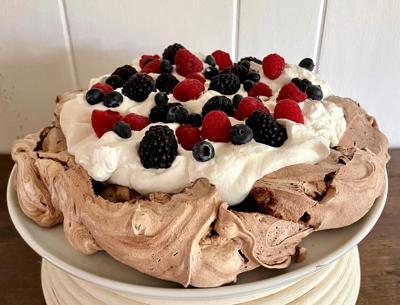In this image, there is a sumptuous dessert displayed on a wooden table with a white, wooden slatted wall as a backdrop. The centerpiece is a creamy, light brown chocolate mousse layered with fluffy white whipped cream, creating a delightful textural contrast. Surrounding the whipped cream is an abundant mix of fresh berries, including blueberries, raspberries, blackberries, and possibly cherries and strawberries, totaling about a cup or two of fruit. The dessert is garnished in a somewhat rustic, unfinished fashion, giving it a homemade yet elegant appeal. This tempting treat is presented on a white plate, which sits atop a small stack of other plates, elevating the dessert and enhancing its visual appeal. The overall setting, including the multi-layered dish pedestal and the wooden table, adds to the warm and inviting presentation of this delectable dessert.